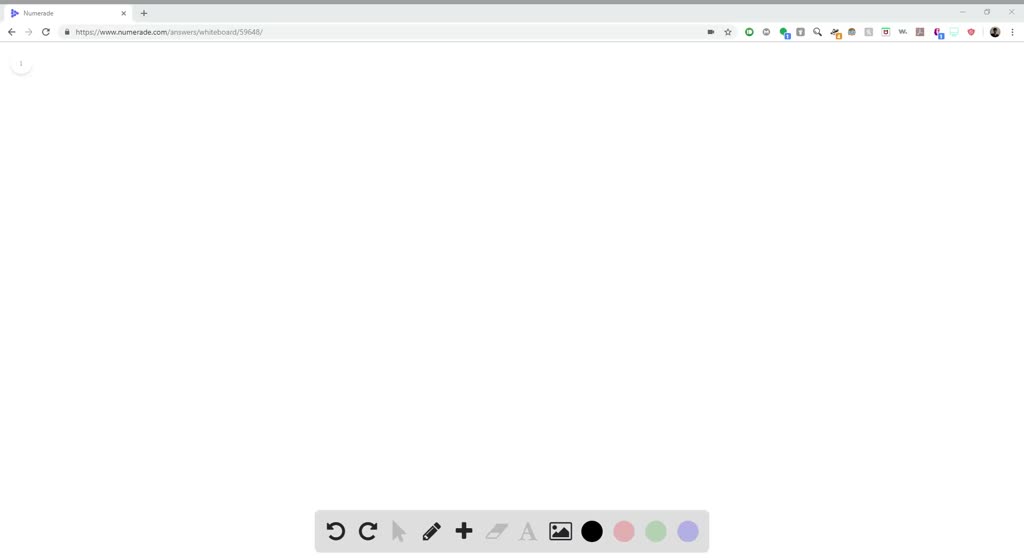A screenshot with a white background captures a web browser interface. The top section of the image showcases multiple open tabs, including an active tab with a website address displayed. On this tab, there is a small profile picture icon adjacent to it. Near the profile picture, there are three vertical dots, possibly two, within a white circle to signify additional options.

Below the address bar, a gray rectangle contains several black icons: a back button, a forward button, and a cursor represented as a gray arrow. Also included are a black pencil icon, a black plus sign, and a letter 'A' in uppercase, appearing in a gray hue.

Further down, the gray rectangle continues to feature a black square icon depicting mountains and a sun, akin to an image placeholder. Surrounding this black square are additional colored circles: one black, one pink, one green, and one purple.